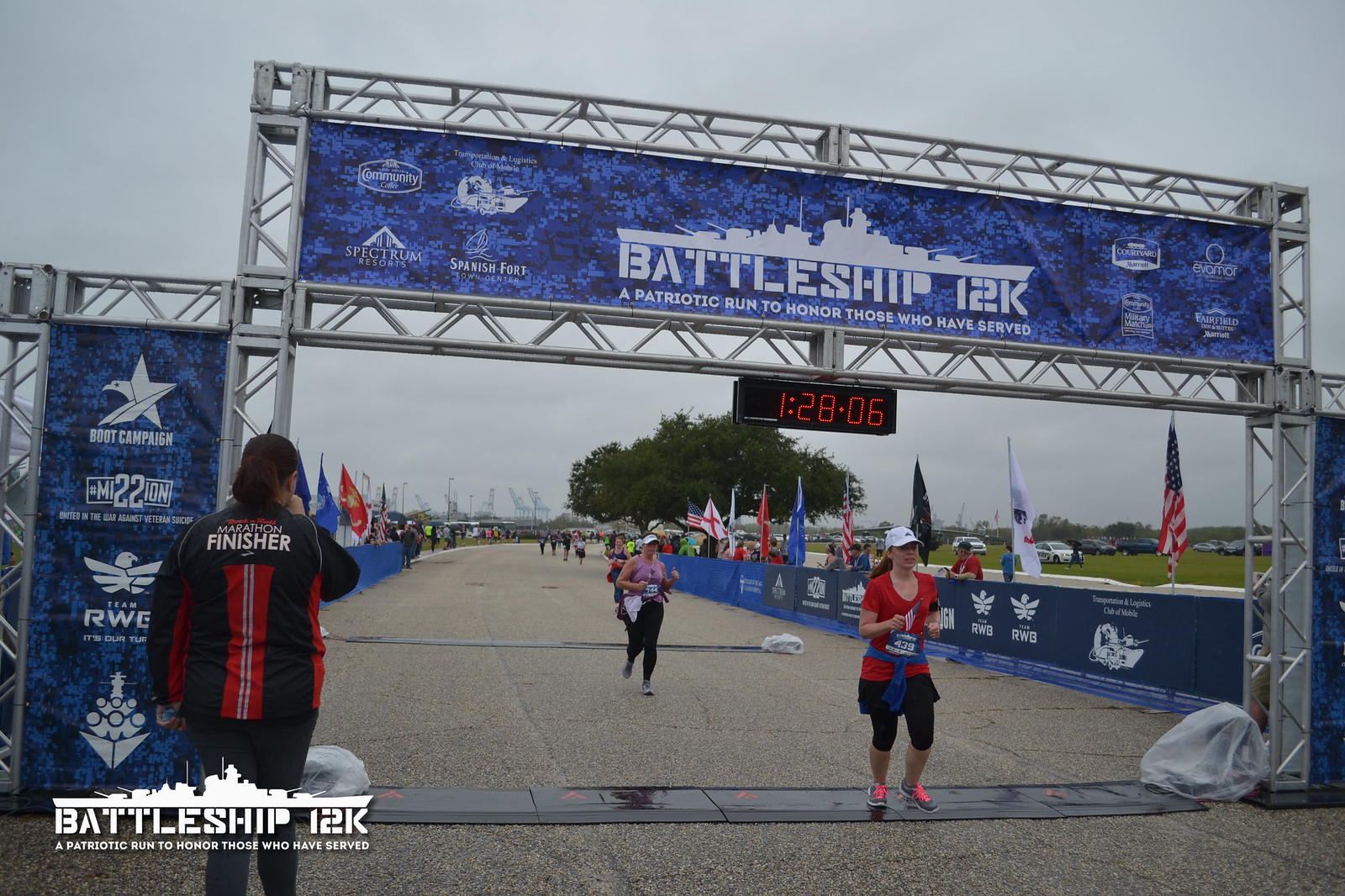This photograph captures the energetic climax of the Battleship 12K, a patriotic run held to honor those who have served. Centered under an archway adorned with a tarpaulin graphic featuring a battleship and the event’s name, “Battleship 12K,” the digital clock above the signage shows the time as 1:28:06. Sponsorship banners from Community Coffee, Transportation and Logistics Club of Mobile, Spectrum Resorts, Spanish Fort Town Center, Marriott Courtyard, Military Match Community, and Fairfield Inn & Suites by Marriott are prominently displayed. 

In the forefront, a woman is crossing the finish line, wearing a red scoop-neck short-sleeve shirt, black leggings, and sneakers with striking pink shoelaces. Her race bib identifies her as number 439. Accompanying her gear is a white baseball cap, further highlighting her athletic attire. In the background, several runners, approximately five or six, are closely following, collectively embodying the spirit of determination and camaraderie that defines the race.